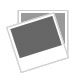The advertisement showcases a premium wood carving chisel positioned vertically in the center of the image. In the top left corner, the company name "SCHAAF" is prominently displayed, with the A's stylized as Delta signs. Below this, it reads "Wood Carving Tools" alongside a logo featuring three circles intersected by a diagonal line. A close-up of the wooden handle is shown beneath, highlighting its detailed grain and craftsmanship, with the caption "Beautiful Ash Wood Handles Provide Excellent Comfort and Balance" in an orangish-brown and black font. The handle itself measures 135 millimeters (5.3 inches). Centrally, the tool's full length is vividly presented, extending 270 millimeters (10.6 inches) with a fine metal blade that tapers to a precise point. In the top right corner, another close-up image focuses on the chisel's sturdy brass ferrule, which is emphasized with the text: "Sturdy Brass Ferrule Protects Handle During Mallet Use."